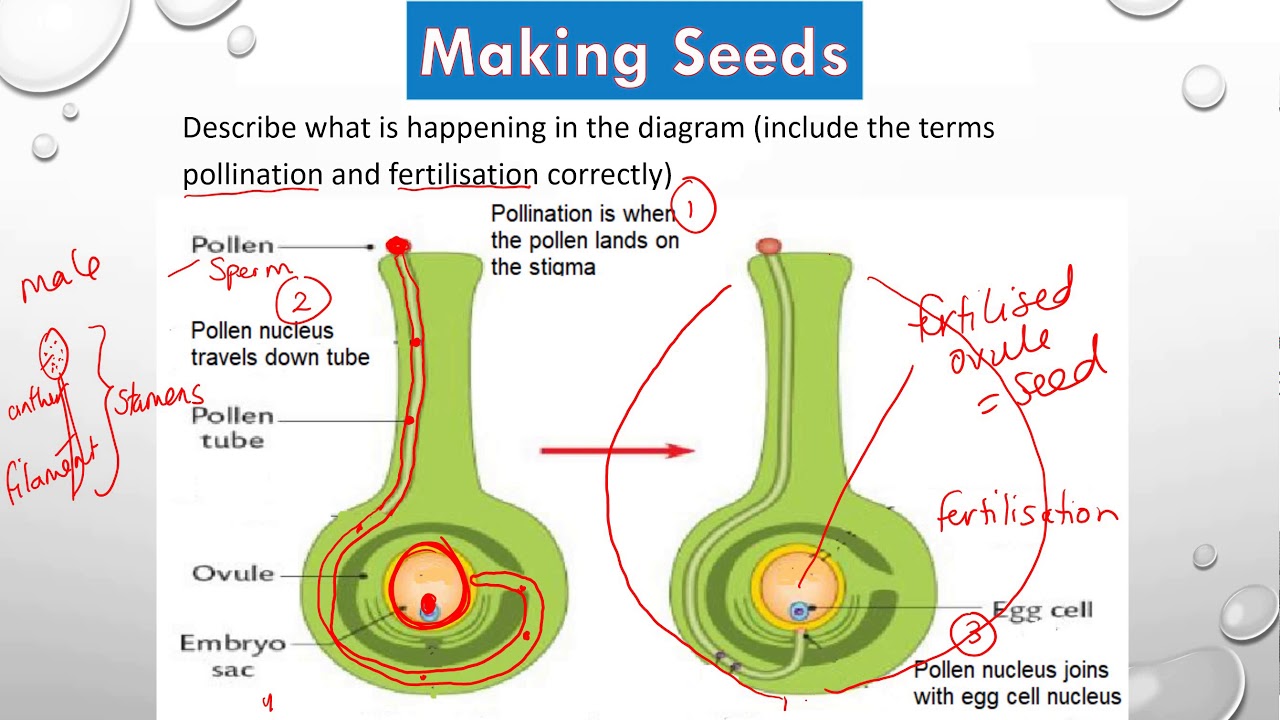This instructional poster, likely suitable for a high school biology class, serves as a detailed guide to understanding the process of seed formation. Titled "Making Seeds," the poster features a dominant blue banner at the top with white lettering. Below, instructions prompt students to "describe what is happening in the diagram, include the terms pollination and fertilization correctly."

The poster displays two main green diagrams resembling genie bottles or vases, set side by side to illustrate different stages of seed development. The diagram on the left, marked with arrows and black text, labels the pollen at the top and the pollen nucleus traveling down a red-drawn tube. The terms "pollen," "sperm," and "pollen nucleus travels down tube" are written near this diagram.

Key annotations in red ink accompany the diagrams, including illegible cursive notations on both sides of the poster. Additional red ink identifies important parts and processes, such as labeling "embryo sac" at the bottom of the left diagram with a distinct red circle and arrow pointing to the corresponding part on the right diagram. This right-hand diagram shows the development state post-fertilization. Red labels also include the word "fertilization," pointing to the area initially marked as the embryo sac, and the label "egg cell" in black text, indicating where the pollen nucleus joins with the egg cell nucleus.

Supporting text in black further explains the process, stating "pollination is when pollen lands on the stigma" at the top of the diagrams, with an underlined red emphasis on "pollination" and "fertilization." Additional red arrows and labels provide clarity, pointing from the pollen nucleus to the egg cell nucleus, culminating in the formation of seeds as encapsulated by the descriptive notations and annotations.

Overall, the comprehensive instructional poster blends both visual aids and detailed text to thoroughly illustrate the critical biological processes of pollination and fertilization leading to seed formation.